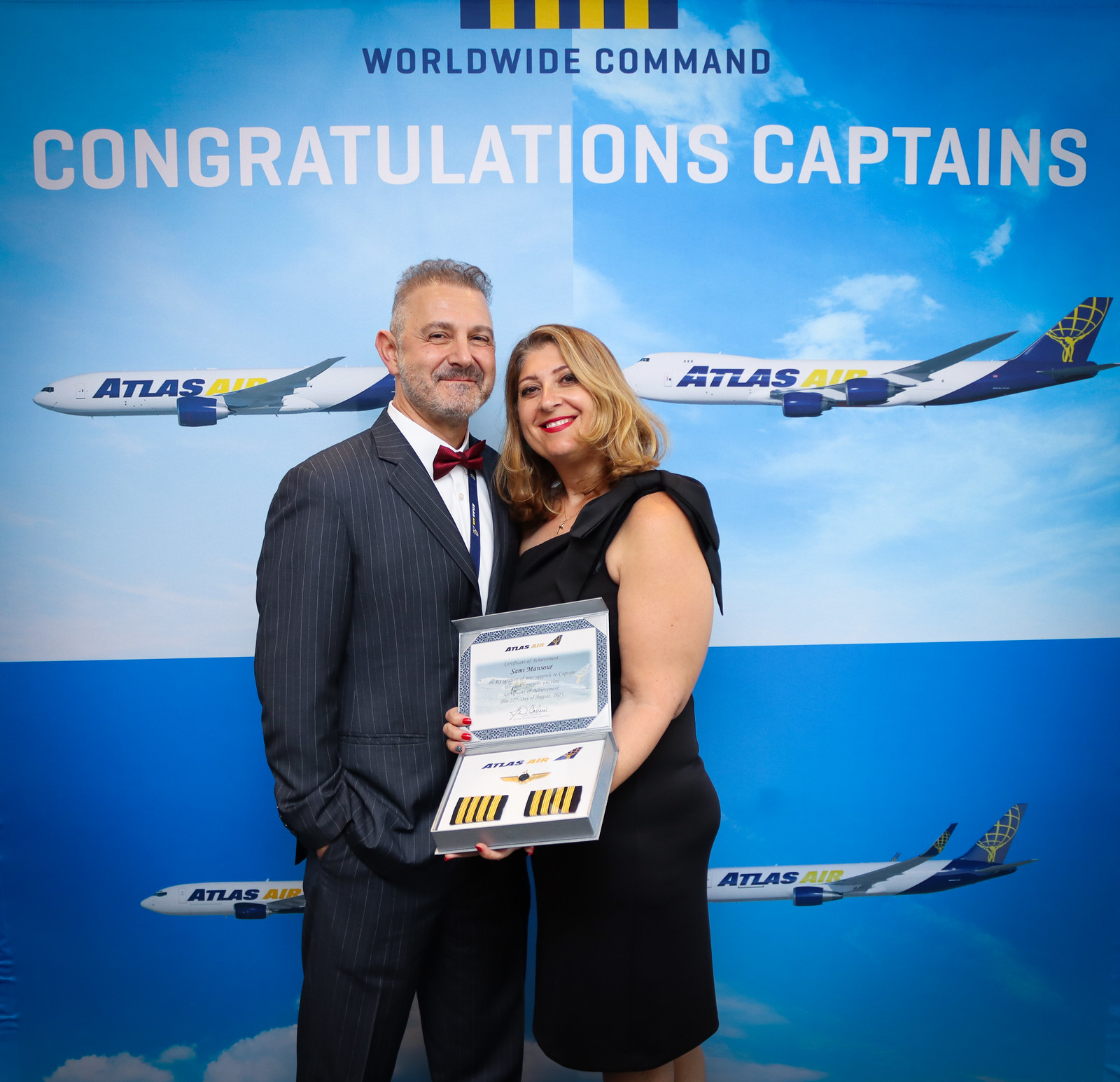In this image, a man and a woman are posing at what appears to be an airline event, possibly a graduation ceremony for captains. The woman, with blonde hair and bright red lipstick, is dressed in a black dress and holding a gray cardboard box that contains an Atlas Air Certificate of Achievement. The certificate bears the name Sammy Mansoor, mentions an upgrade to captain, and is dated August 22, 2023. The man is wearing a blue pinstripe suit with a burgundy bow tie, a white dress shirt, and he has a beard and mustache. Behind them is a banner with blue and white text that reads "Worldwide Command, Congratulations Captains." The background also features a wallpaper depicting four airplanes in mid-flight with blue and yellow text "Atlas Air" on their sides. Both individuals are smiling, marking this celebratory moment.